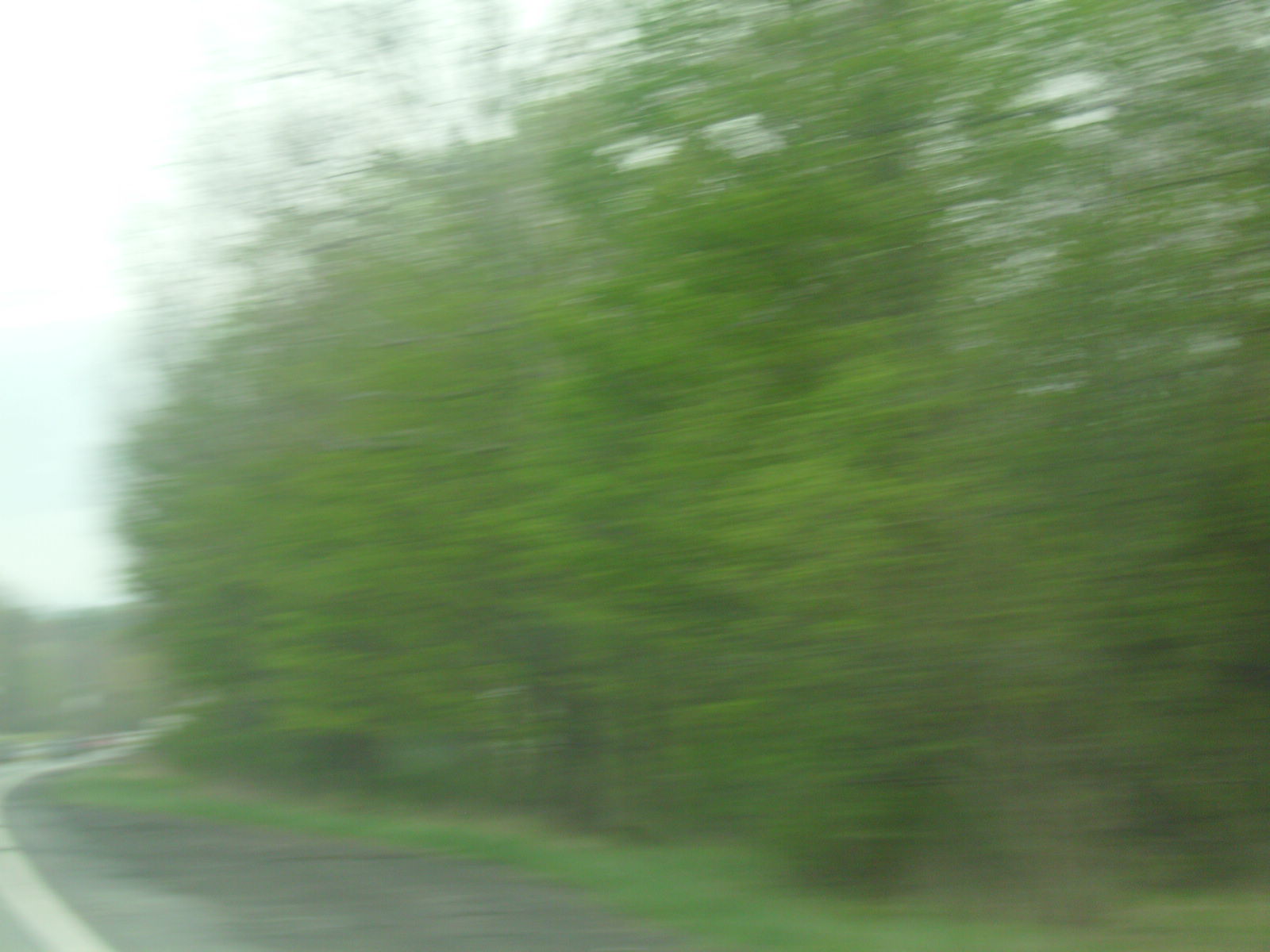The image is a very blurry outdoor photograph capturing a wooded area that transitions into a roadway. On the left side, the sky appears blue at the bottom fading to white as it ascends. The upper left corner prominently features this sky transitioning to a cloudy gray. Spanning from the center to the right, a variety of trees in different shades of green fill the scene, creating a forested backdrop with some spacing that allows glimpses of the sky. The ground beneath these trees consists of green grass and patches of dark brown to almost black dirt. A road emerges at the bottom left of the image, marked by a distinct white stripe indicating the edge of the pavement. This stripe curves gently into the distance, giving the impression that the roadway meanders through the natural setting. In the far background, there is a hint of a mountainous region, characterized by brown with some greenery.